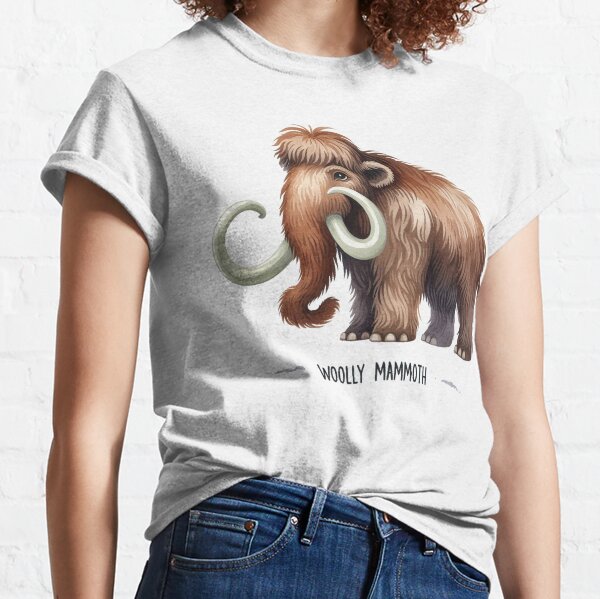This image illustrates a young woman standing against a white brick wall, wearing a slightly off-white t-shirt that features an eye-catching, cartoon-style woolly mammoth graphic. The mammoth is a rich combination of browns and tans, sporting large white tusks and a tuft of long fur resembling a bowl cut on its head. Below the mammoth illustration, the text "WOOLLY MAMMOTH" is clearly printed in black letters. The woman is dressed in blue denim jeans, with the front part of her t-shirt casually tucked in, and the sleeves are rolled up slightly. Her curly, reddish-brown hair is partly visible, cascading to just under her shoulders. She has medium-light skin and stands with her arms relaxed at her sides, making the t-shirt and its unique design the focal point of the composition, suggesting it is likely an advertisement for the apparel.